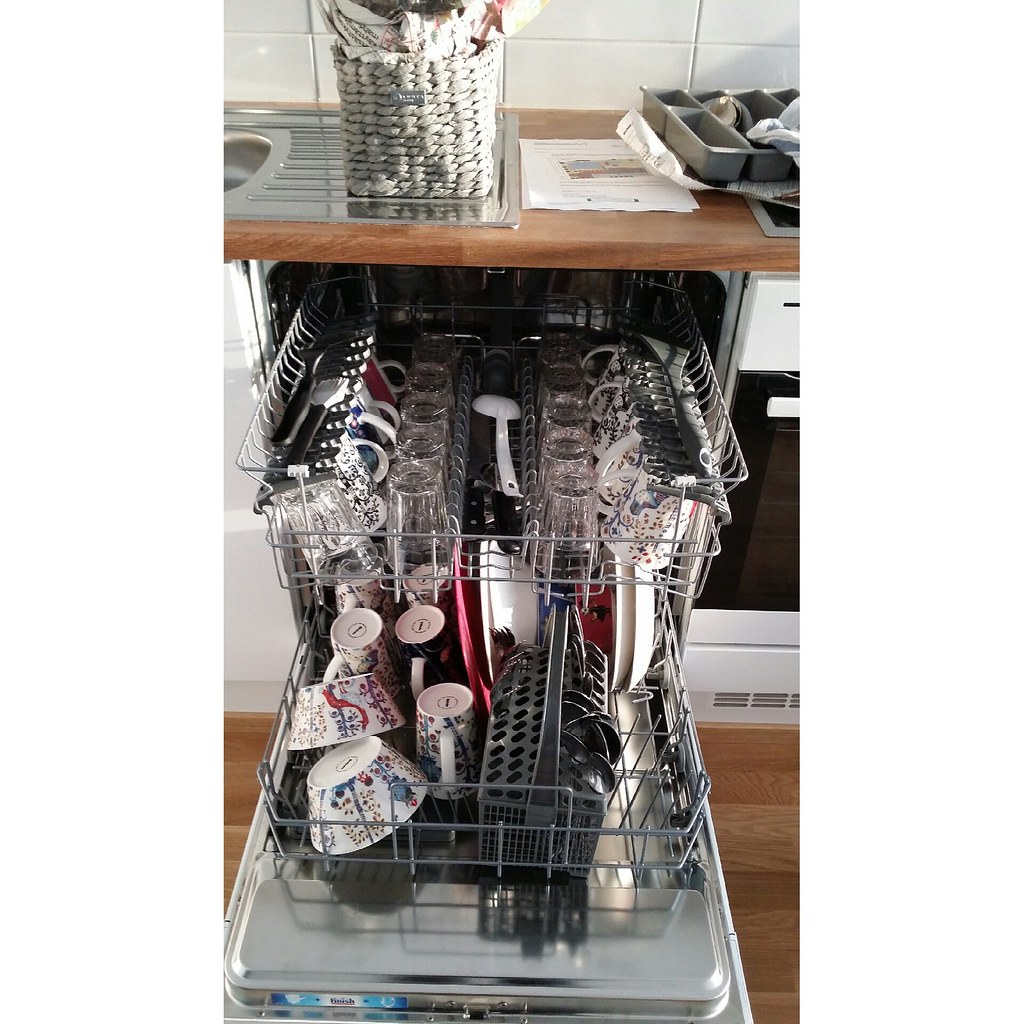The image depicts a kitchen scene centered on an open dishwasher loaded with various dishes. The hardwood floor extends throughout the kitchen, partially visible on the right side where a type of plant can be seen. The dishwasher is filled with a diverse array of items. On the top rack, clear and white glasses are organized in the glass holders, while ceramic mugs with black designs and medium-length glasses with white ceramic designs are placed alongside. The bottom rack houses several bowls with varying depths and five cups, with the utensils stored in the gray rolling rack on the right side. Additionally, there are plates positioned at the back of the dishwasher, and some knives and spoons in the silverware holder positioned in the center. Above the dishwasher, a wooden countertop is visible, featuring a white basket, a gray container, and a sheet of paper. To the left of the dishwasher, part of a silver stove can be seen, further enhancing the detailed and homey kitchen atmosphere.